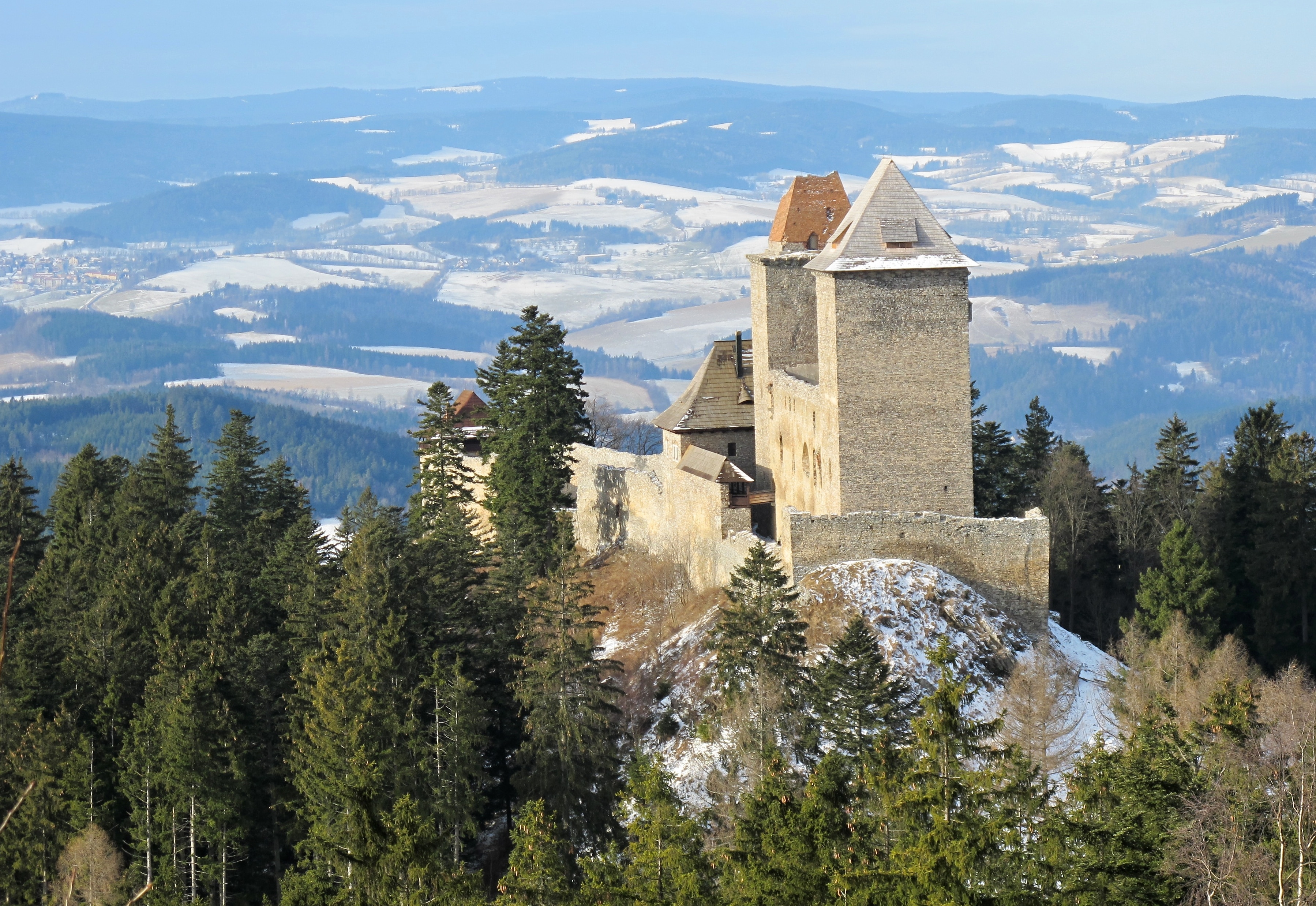This horizontal rectangular photograph, likely taken from an aerial perspective, showcases a potentially abandoned stone building perched on the crest of a snow-covered mountain, possibly in the Alps. The structure, which appears to be a castle, has a distinctive Germanic architectural style with squared-off features and Bavarian-style roofs. The tan or light brown stone of the building, partially in ruins, includes two towers with pointy roofs and some sections without a roof, exposing the interior. A wall surrounds the building, which is nestled amid dense evergreen trees. The scene captures the striking contrast of snow on the ground and the trees, and also reveals lower elevations where snow blankets the valleys. Overall, the image is framed by a clear, blue sky with a few clouds, highlighting the breathtaking height and vantage point of the castle.